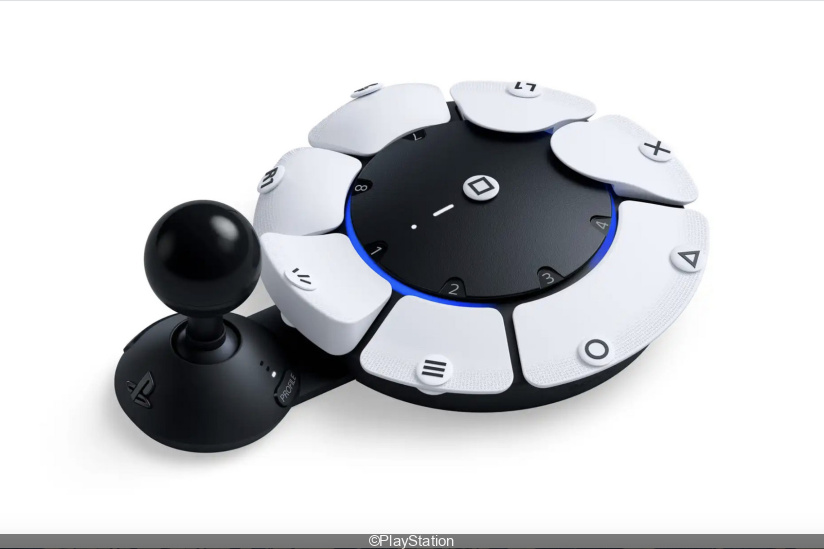The image depicts a futuristic PlayStation controller set against a plain white background, complete with a Copyright PlayStation watermark at the bottom. The controller itself features a unique circular shape with various buttons positioned around the outer edge, resembling a spacecraft or a turtle shell with a distinctive "head." The outer ring of buttons includes recognizable symbols such as O, triangle, X, L1, R1, and three spread-out horizontal lines. These buttons are white with black symbols. 

In the center of the circle is another black ring, marked with the numbers 1 through 8. There’s also a white button with a square symbol, connected by a white line to one of the larger paddle buttons on the outer ring. A black joystick, complete with the PlayStation logo, extends from the structure on a black arm, resembling an old-school arcade joystick or a car shifter. Blue lights peep intermittently from between the segments of the black and white sections, adding an intricate glow to the design. Although its exact function is unclear, this intricate and modern-looking device inspires curiosity and awe.